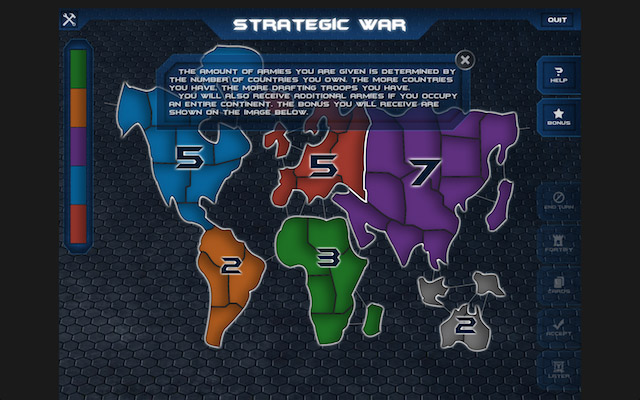The image depicts a colorful, cartoonish map titled "Strategic War," set against a black background adorned with a subtle honeycomb pattern. The map itself is divided into numbered and color-coded zones representing different continents: North America (blue, 5), South America (orange, 2), Europe (red, 5), Africa (green, 3), Asia (purple, 7), and Australia along with surrounding areas (gray, 2). At the top of the image, bold white text reads "Strategic War," followed by a detailed paragraph explaining the game mechanics: "The amount of armies you are given is determined by the number of countries you own. The more countries you have, the more drafting troops you have. You will also receive additional armies if you occupy an entire continent. The bonuses you will receive are shown on the image below." On the right side of the screen, there is a small vertical menu with options labeled "Quit," "Help," and "Bonus." The overall style combines elements of digital graphic design, likely indicating that the map is from a video game or a digital board game.